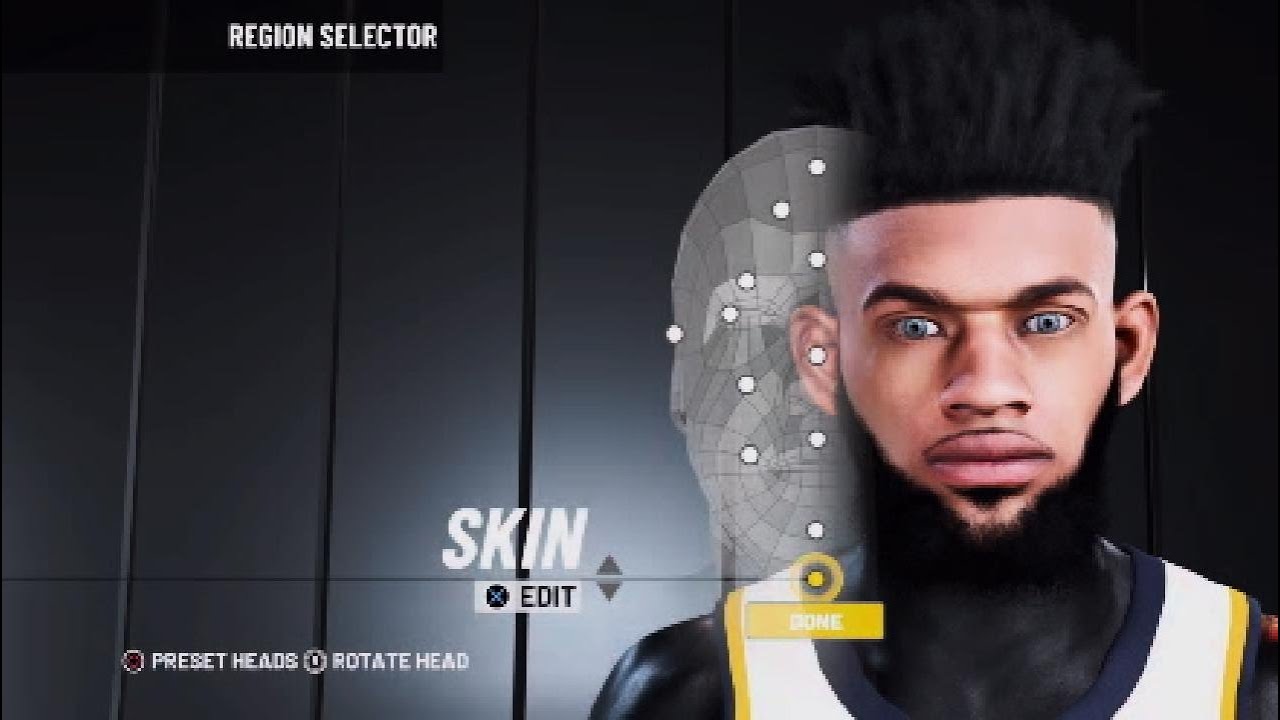The image appears to be a screenshot from a video game, featuring a character customization screen. At the top of the screen, white text on a dark background reads "Region Selector." Toward the bottom, the options "Skin" and "Edit" are visible, suggesting that this section allows for modifications to the character's appearance. 

In the center, there's a digital representation of a male character who appears to be African-American with closely resembling realistic human features. The character has black hair, subtle blue-gray eyes which might also have brown tones, and distinct facial features including a wide nose and a mixture of facial hair. His facial hair consists of a thin mustache paired with a goatee that extends to his ears. 

He is dressed in a jersey with a color scheme of white, yellow, and black. The background behind the character also appears to be digitally rendered, aligning with the overall video game environment. Additionally, options like a preset head and a head rotation feature are present, indicating the user can fine-tune the character's facial characteristics.